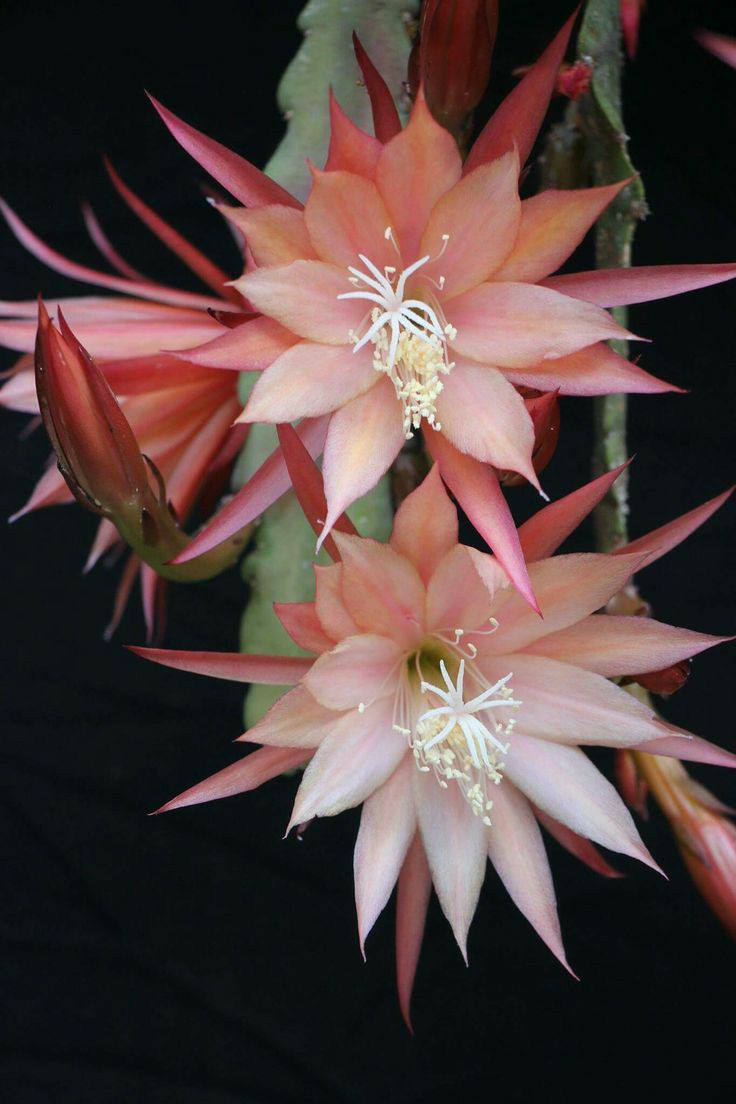This photograph captures three stages of a cactus flower: two fully bloomed flowers and a prominent bud. The background is a stark black, drawing attention to the delicate details. At the center, a ridged green cactus surface serves as the base from which the flowers emerge. The two main flowers face the viewer directly, showcasing layers of pointy petals. The topmost petals are a pale pink, with slightly darker pink and orange hues filling the layers behind. Each flower's center features intricate details: star-shaped white tendrils and clusters of thin stems capped with tiny white pieces, likely for pollination. To the left, another bloomed flower is visible from the side, echoing the same multi-layered petal structure. Nestled between the two main flowers is a striking bud, resembling a piece of asparagus with a vividly pink tip poised to bloom.